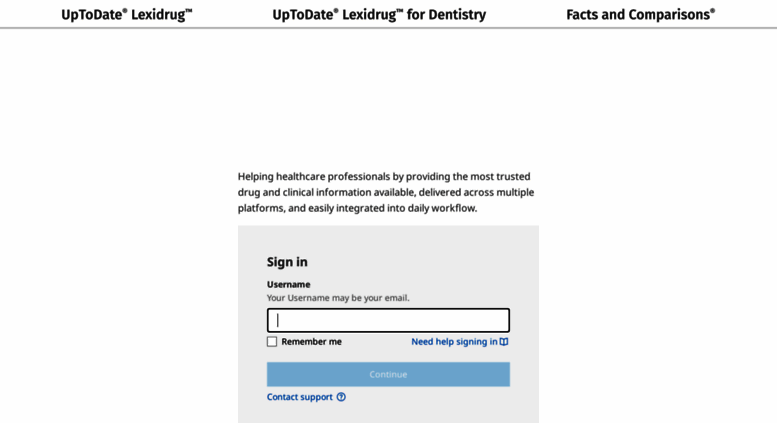This cropped screenshot captures a section of the Lexidrug website, a medical platform dedicated to medication research. Set against a white background, the screenshot displays three horizontally listed categories at the top. On the top left, the category reads "Up to Date Lexidrug," the center features "Up to Date Lexidrug for Dentistry," and on the right, it says "Facts and Comparisons." A thin gray line runs beneath these categories.

Toward the bottom of the screenshot, a small paragraph in light gray letters is centered, stating, "Helping Healthcare Professionals by Providing the Most Trusted Drug and Clinical Information Available, Delivered Across Multiple Platforms and Easily Integrated into Daily Workflow."

Below the paragraph, a gray login box can be seen. The top left of this box features the bold black text "Sign In." Directly below this, the label "Username" appears in smaller black letters, accompanied by a large text box for the username input. On the bottom left of this text box, a small square checkbox labeled "Remember Me" is visible. To the right of this text box, the hyperlinked text "Need Help Signing In?" appears in blue. Below these elements, a large "Continue" button is present but is unclickable, appearing gray.

Further down, on the bottom left of the gray box area, the text "Contact Support" is displayed. At the very bottom, two horizontal lines are centered, with the word "OR" placed between them in small black letters. The screenshot is cropped off just below this point.

This descriptive caption provides a detailed overview of the elements present in the captured section of the Lexidrug website.